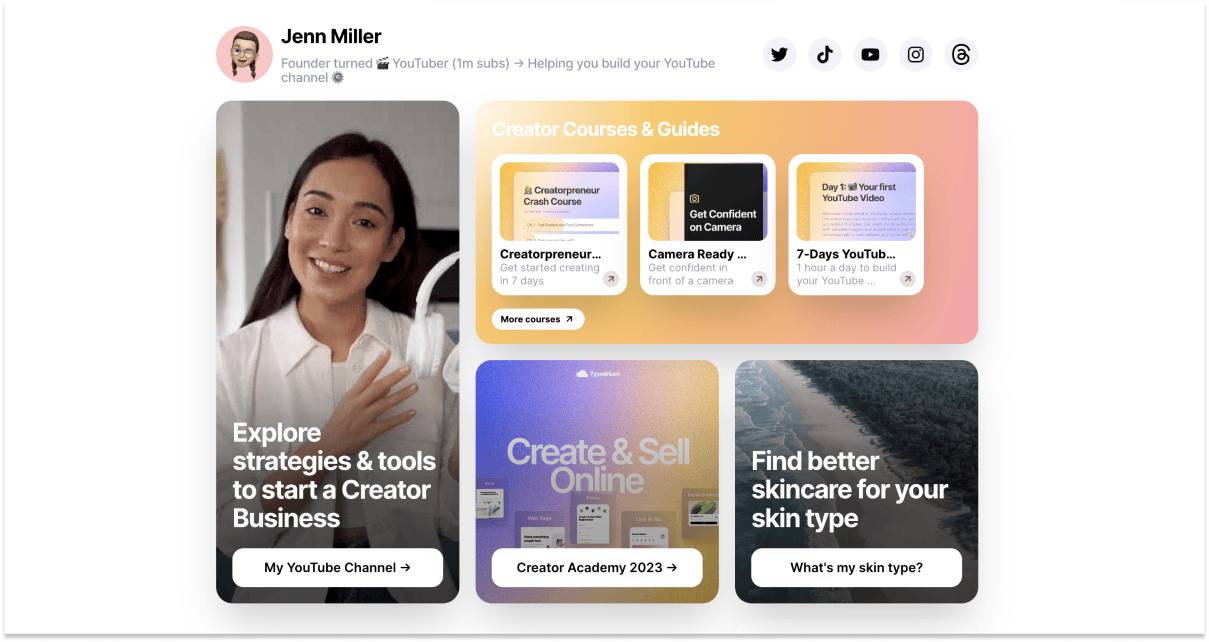This image, presumably from a social media platform, prominently features Jen Miller. Her name is displayed in black text with a small, round profile picture to the left. The picture has a pink background and shows an avatar of Jen sporting glasses and two pigtails. Below her name, it reads "Founder turned YouTuber (1 million subs)" followed by a right arrow and the phrase "helping you build your YouTube channel."

The main visual element is a square image of a woman with long black hair, wearing a white, long-sleeved button-down blouse and a white undershirt, holding a white headset. Overlaid text in white says, "Explore strategies and tools to start a creator business." Below this image, a white speech bubble contains the text "My YouTube channel" with a black right arrow.

At the top of the image, the background transitions from yellow to pink peach, with white text reading "Creator courses and guides." Below, there are three small squares:

1. "Create Her Preneurship: Get started creating in 7 days"
2. "Camera Ready"
3. "Seven Days YouTube"

Additionally, there are more course offerings in two more boxes:

1. "Create and Sell Online: Creator Academy 2023"
2. "Find Better Skincare for Your Skin Type," accompanied by a small box saying, "What's my skin type?"